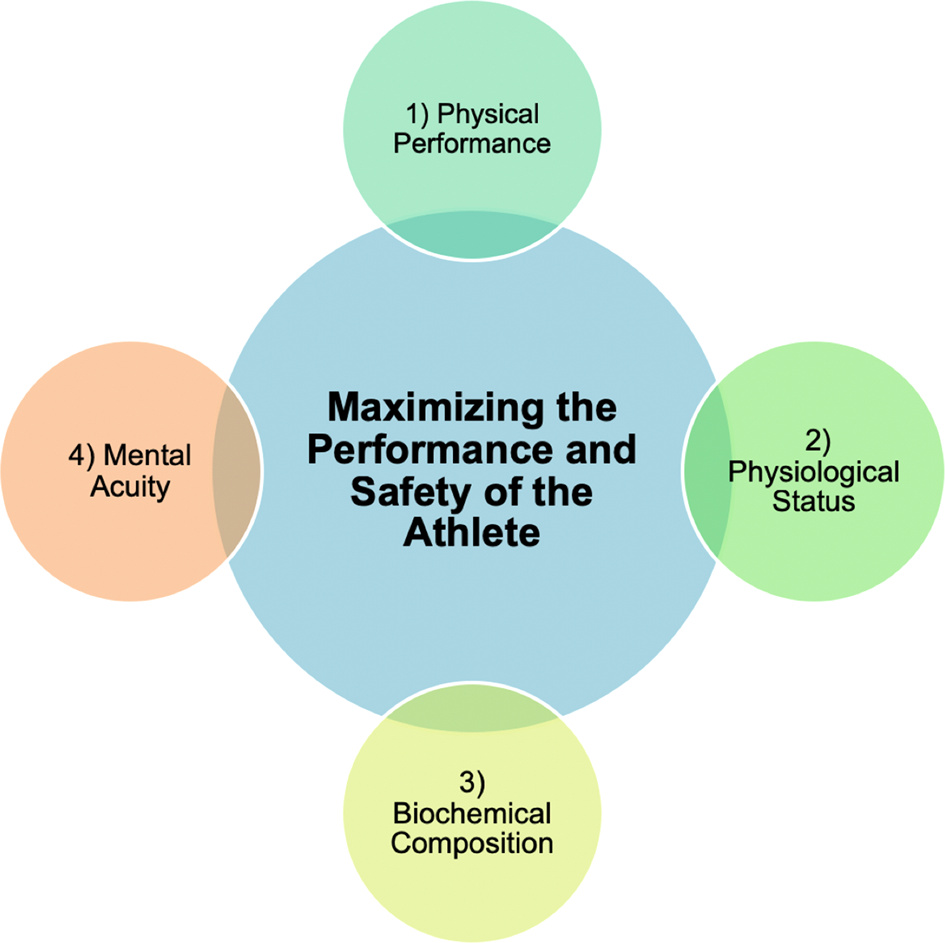This detailed diagram illustrates a central blue circle surrounded by four smaller overlapping circles positioned at each cardinal point: north, south, east, and west. The central blue circle prominently displays the text "Maximizing the Performance and Safety of the Athlete" in black. Each overlapping circle addresses a specific aspect of athletic enhancement. At the north position, the first circle, labeled "1," includes the text "Physical Performance." To the east, the second circle, labeled "2," reads "Physiological Status." The southern position features a yellow circle, labeled "3," with the text "Biochemical Composition." Finally, the western circle, labeled "4," bears the text "Mental Acuity." Each of these aspects interacts with the core concept in the central circle, emphasizing a holistic approach to enhancing an athlete's capability and well-being.